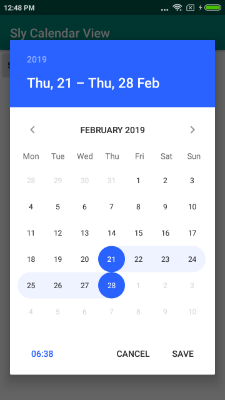**Caption:**

A smartphone screen displaying a grayed-out page behind a prominent pop-up window is shown. The device indicates it is 12:46 PM with a full battery. The underlying screen partially visible offers a slide calendar view with significant empty space below. The pop-up box, featuring a blue border at the top, highlights the period of Thursday, February 21st to Thursday, February 28th, 2019. In its center, large bold black capital letters state "February 2019," flanked by left and right arrows. Below, the days of the week are listed: Monday through Sunday. The calendar grid reveals February starting on a Friday and ending on the 28th, a Thursday. The overlap includes the last four days of January and the first ten days of March. At the bottom left in blue text, it reads "06:3A," while the bottom right shows options in black capital letters: "CANCEL" and "SAVE."